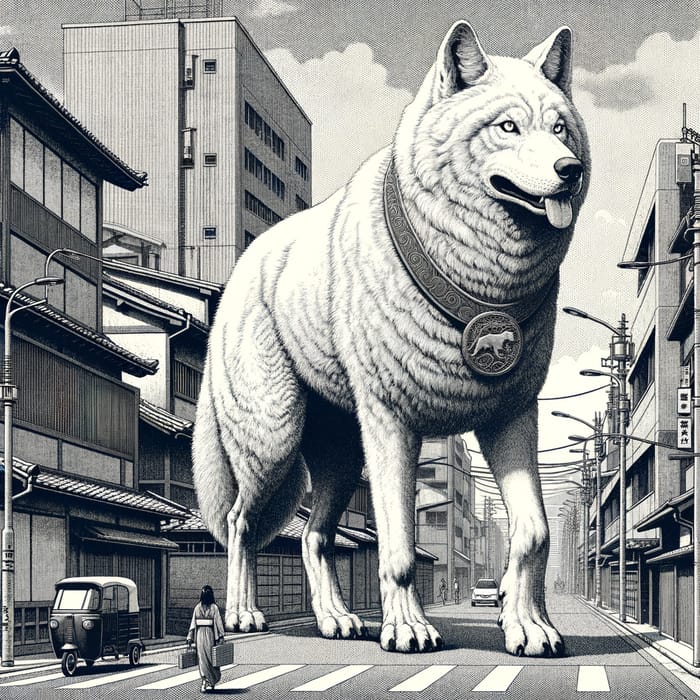This black and white image, likely an ink drawing from an anime or manga, portrays a bustling city street with Asian-style architecture. Dominating the scene is a colossal, well-groomed husky-like dog, about three to five stories tall, with its four paws firmly planted on the ground. The dog, possibly symbolizing a mythical deity, has its tongue out and is gazing slightly to the right. It wears an ornate metallic collar featuring a circular medallion adorned with the image of an animal, possibly a ferret or mongoose.

In the foreground, an Asian woman in a kimono walks toward the dog, carrying two suitcases and crossing a pedestrian walkway. To her left, a small tricycle-like vehicle, common in Southeast Asia, is parked, while a car is positioned behind the dog's massive paw. The scene includes numerous streetlights, power lines, and signs with vertical Asian characters, all beneath a cloudy sky. Despite the detailed urban setting, there are only a few other people visible in the distance, emphasizing the surreal scale of the giant dog against the city's backdrop.